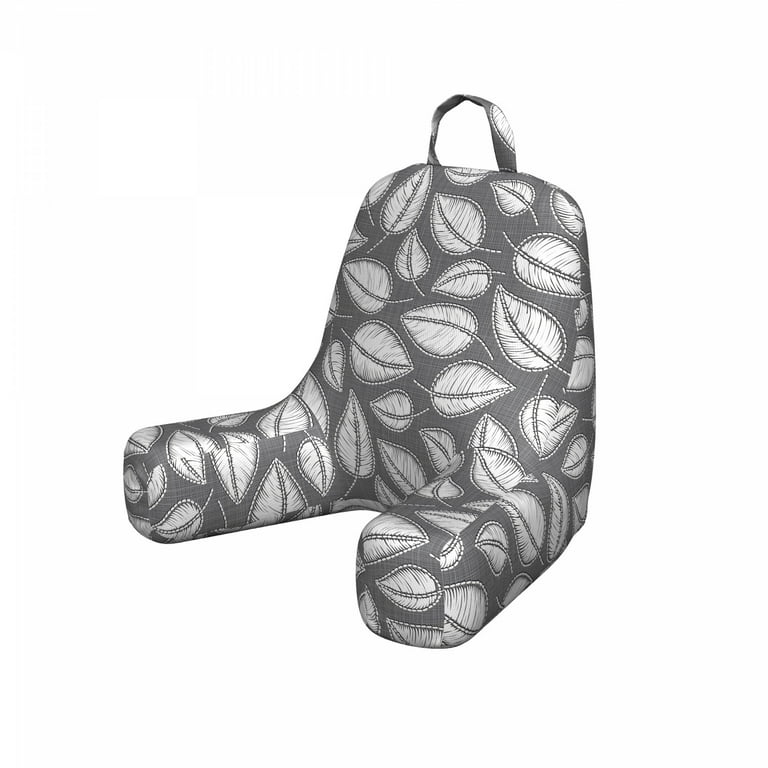The image depicts a floor chair or backrest pillow, likely featured in a product catalog due to its isolated, white background. The chair has a plush, beanbag-like structure, designed for supporting the back while seated on the floor or in bed. It features two extended armrests providing additional support and comfort. The fabric is a gray tweed with an intricate pattern of white leaves, each leaf detailed with a vein running through the middle and varying in size and shape, giving an artistic, sketched appearance. The top of the chair has a functional handle made from the same fabric, allowing for easy portability. This functional and stylish chair is well-suited for lounging, reading, or providing support for a baby learning to sit up.